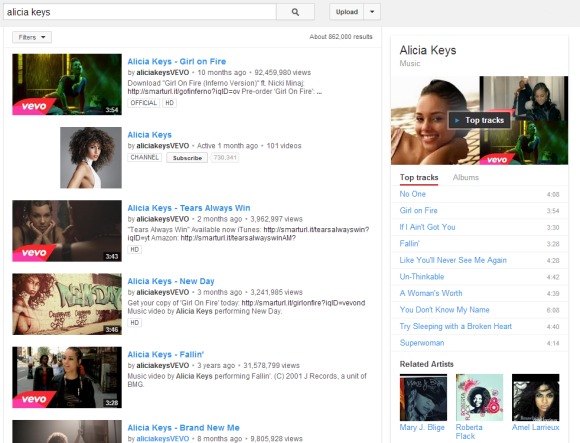This screenshot showcases a web search page with a white background, divided into two primary columns. The overall design is framed within a large square shape. At the very top of the page, a gray border spans the entire width, encapsulating a white search box on the left where the term "Alicia Keys" has been entered. Adjacent to this search box is an upload button.

Directly below the search box is a button with a drop-down menu, likely for filtering search results. A text in this section indicates approximately 86,000 results. The main content area below this comprises two distinct columns against a predominantly white backdrop.

The left column displays six different search results related to Alicia Keys. Each result follows a uniform structure; a thumbnail image on the left (the first one appears to be from Vevo and includes a time stamp), accompanied by a title such as "Alicia Keys - Girl on Fire," and other relevant details including view counts, leading to specific webpages.

The right column focuses on Alicia Keys herself, featuring her name, a brief descriptor ("Music"), and several photographs. It lists her top tracks with clickable links, presumably redirecting users to pages with more detailed information. Additionally, this column includes a section for related artists.

In summary, the search engine interface features a simplified, two-column layout: the left dedicated to search result thumbnails and text, and the right offering specialized information about Alicia Keys and related content.